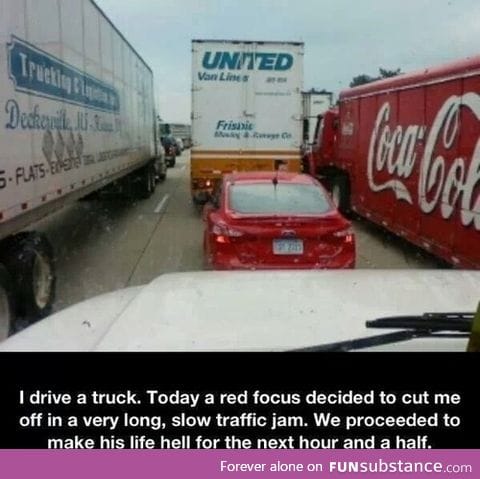This compelling image, captured through the windshield of a truck, vividly depicts a severe traffic jam on a three-lane highway. The photograph shows a red Ford Focus sedan trapped and surrounded by large vehicles from all sides. Positioned to the left is a white tractor-trailer, while to the right, there's a prominent red Coca-Cola truck. In front of the Focus is a United Van Lines semi-truck, easily identifiable with its distinct blue and orange branding. Directly behind the red Focus, in the foreground of the image, we see the white hood of the truck from which this photo is taken.

The scene portrays a moment of frustration and retribution as the trucks box in the small red sedan, effectively "sandwiching" it with nowhere to escape. The colors in the image are dominated by blue, white, red, and splashes of gray and pink, emphasizing the commercial nature of the surrounding trucks. The descriptive text at the bottom of the image, displayed in white font on a black bar with a subsequent pink bar, reads: "I drive a truck. Today, a red Focus decided to cut me off in a very long, slow traffic jam. We proceeded to make his life hell for the next hour and a half." The image appears to be styled as a meme and is credited at the bottom with "Forever Alone on funsubstance.com," suggesting it is intended for circulation on social media, highlighting a common frustration among truck drivers.